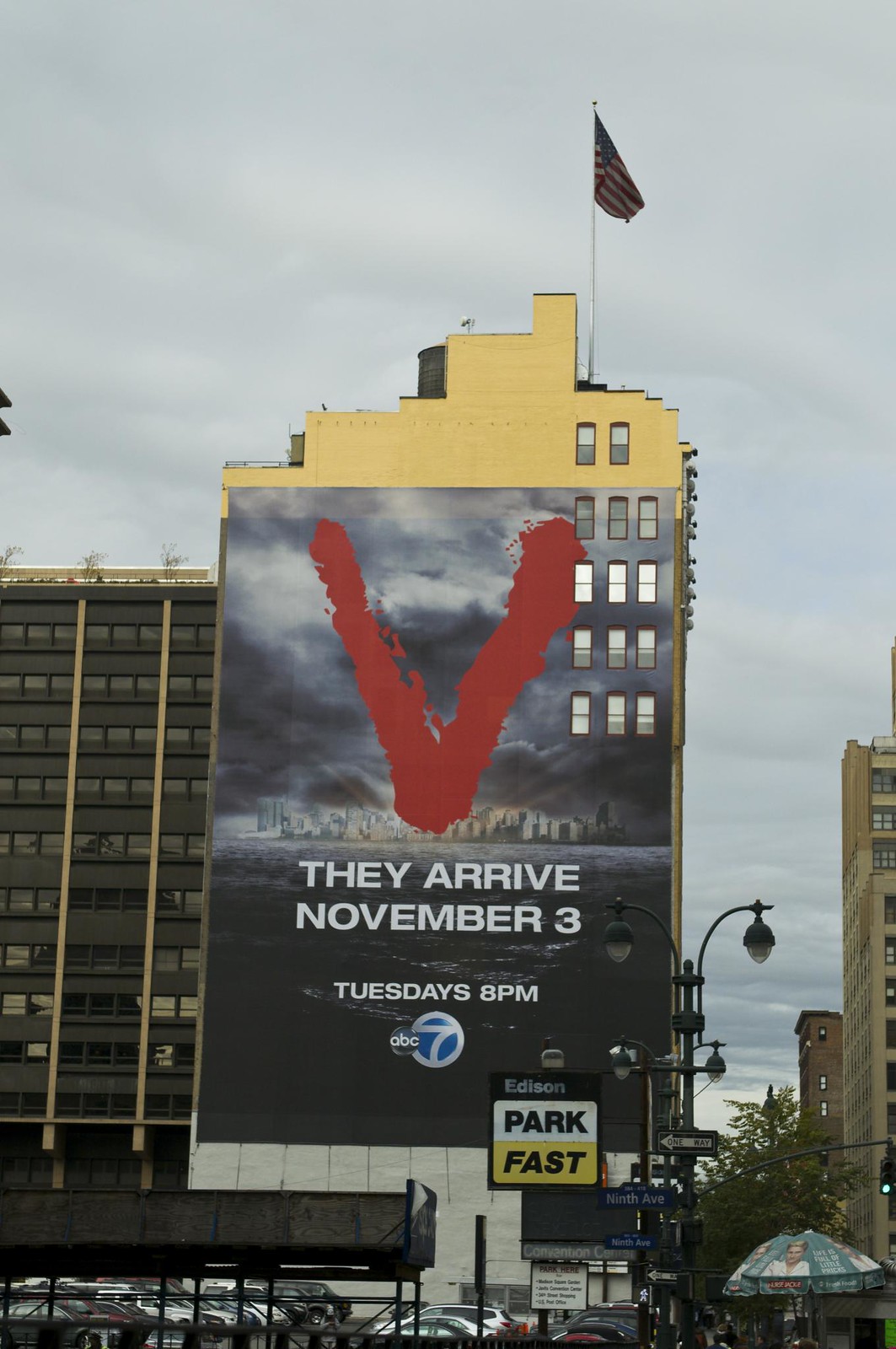The image captures a tall, yellow-tan building featuring a prominent advertisement on its side, mainly adorned with a striking red "V" at the top. This large mural, a promotion for a TV show airing on ABC, occupies almost the entire side of the building, obscuring 12 windows. Below the "V," set against a backdrop of dark storm clouds, is a city skyline that appears to represent a coastal metropolis like New York City, with blue and black colored water depicted beneath it. The ad announces "They arrived November 3, Tuesdays 8 p.m. ABC," accompanied by the ABC Circle 7 logo.

Above the massive painting, two more windows are visible, and an American flag flutters against the overcast sky. To the building's left, a neighboring structure is partly visible, marked by rows of windows, while on the right, at street level, there's a parking lot with a sign reading "Edison Park Fast." The lot is populated with cars, and nearby, an umbrella featuring a woman's face is visible, hinting at the presence of a food cart or similar vendor. Surrounding the scene are streetlights, traffic signs, and additional city buildings, contributing to the dynamic urban atmosphere.